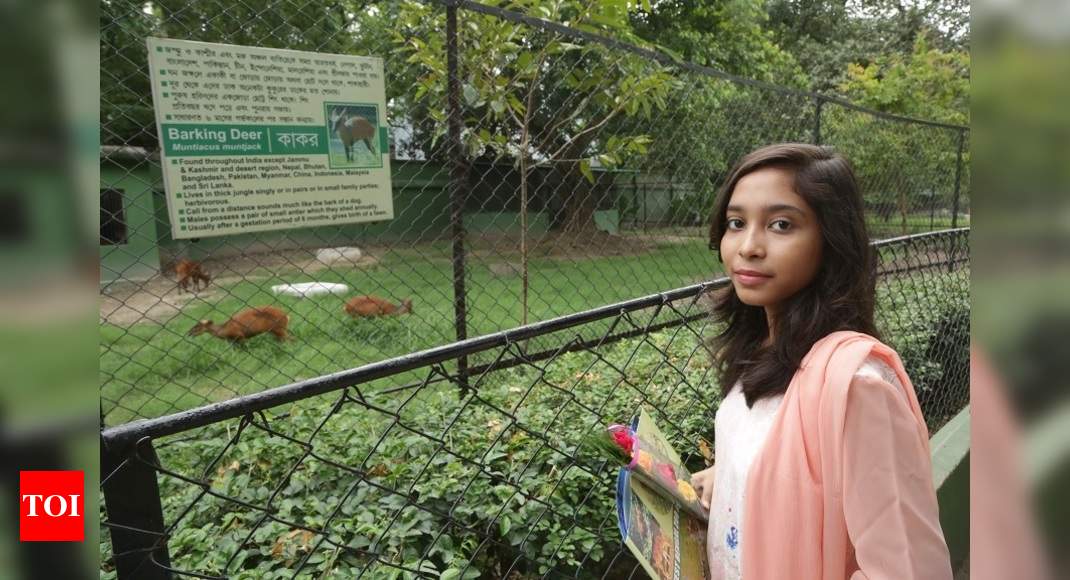In the foreground, a young girl with dark hair stands in front of a fence, wearing a pink jacket and a pink shirt. She holds a magazine or brochure in one hand and possibly a snack in the other. Behind her, there's a shorter chest-high fence with a bush growing beside it. Beyond the bush, a taller fence encloses an area containing several barking deer grazing in a lush field. The enclosure also features a green building and is dotted with trees. A sign on the fence reads "Barking Deer," accompanied by text in English and possibly another language, along with an illustrative picture of the deer. A red square logo with the letters "TOI" in white is visible in the bottom left corner of the sign. This scene appears to be set in a zoo or animal preserve.